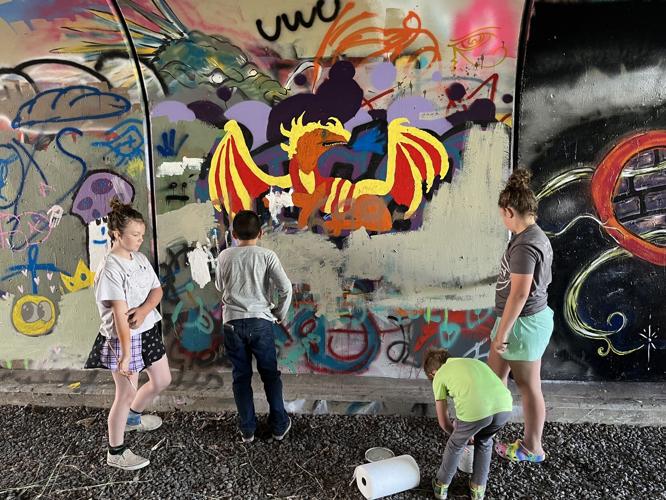The photograph captures a scene of four children, two boys and two girls, all standing on a gravel floor in front of a graffiti-covered wall. The top three-fourths of the image is dominated by the wall, which is adorned with various colorful graffiti, prominently featuring a dragon with yellow and red wings and brown skin in the middle. The bottom fourth of the image shows the children, who appear to be Caucasian, two on the left and two on the right, with a roll of paper towels placed on the ground between them. One child looks like they are bending over a paint can, possibly suggesting they are either adding to the graffiti or cleaning it off. The setting feels open and public, hinting that the kids might be engaging in some form of street art or maintenance. The scene is vibrant with colors like gray, red, yellow, orange, purple, black, blue, and pink, adding to the dynamic feel of the activity taking place.